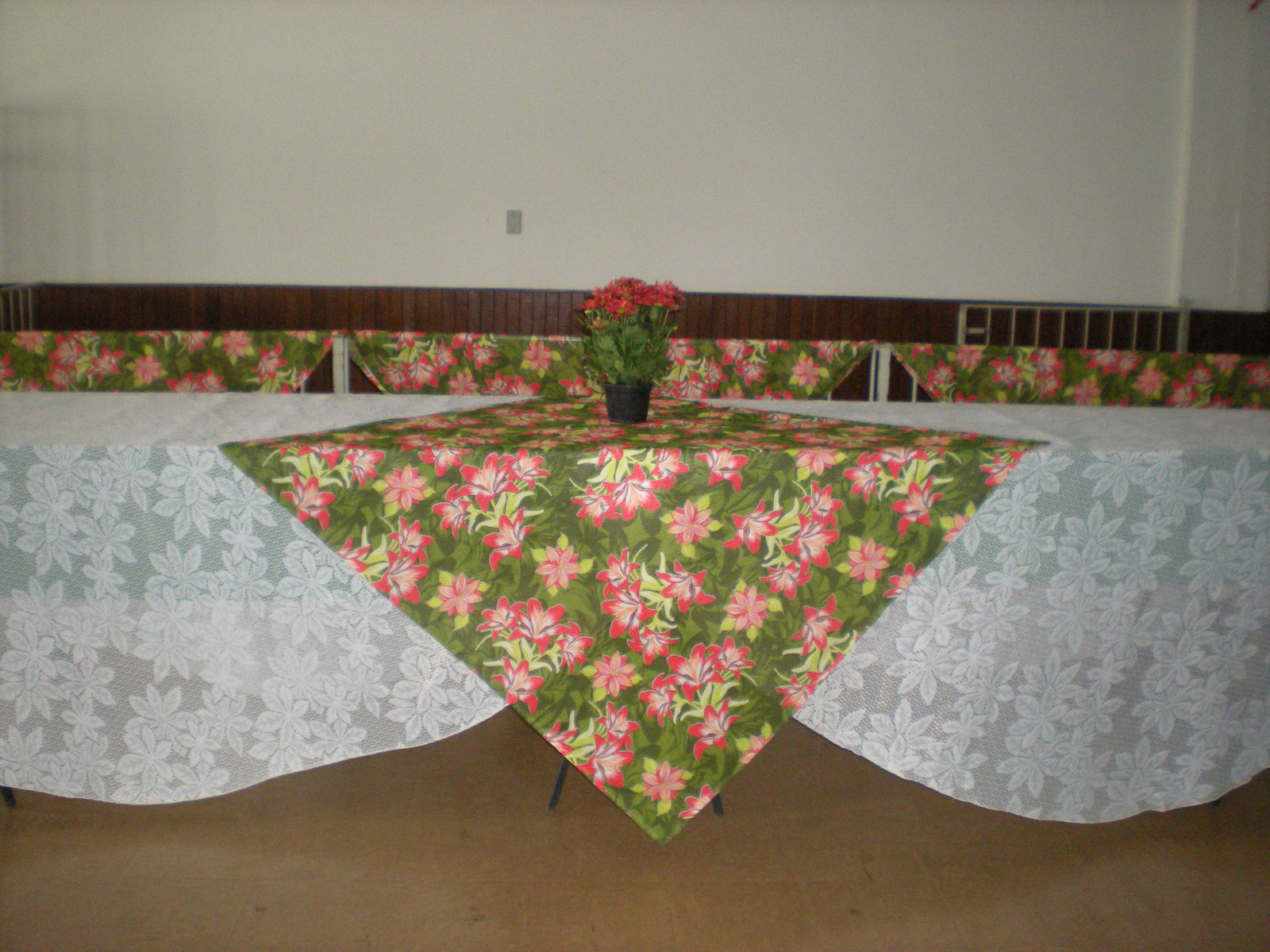The color photograph captures a banquet-like setup featuring two rows of tables, with one row positioned against a wooden wainscoted wall with an off-white painted upper section, which is detailed with a visible light switch. The tables are adorned with large white lace tablecloths that extend far past the table edges, creating a draped effect. In addition to the lace, a diamond-shaped tablecloth with a green background, red flowers, and lighter green leaves is artistically folded and draped over the white lace, contributing a splash of color and pattern to the scene. There is also a similar tablecloth covering the seating area. Central to the tables is a black planter brimming with vibrant reddish-pink flowers, resembling chrysanthemums, and lush green leaves. The arrangement is elegant, with floral motifs and color coordination enhancing the visual appeal.